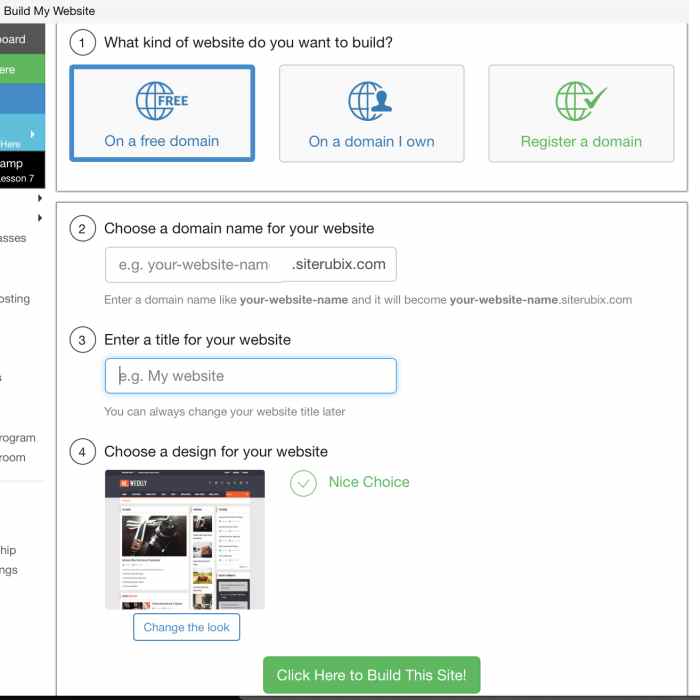The image is a screenshot of the "Build My Website" page on a website. At the very top, there is a horizontal gray bar with the text "Build My Website" in black on the left-hand side. Below this gray bar, there are several colorful bars stacked vertically on the left side. From top to bottom, the bars are gray, green, blue, light blue, and black.

On the right side of the image, the header text reads, "What type of website do you want to build?" Below this header, there are three options: 

1. "On a free domain" - This option has a sphere icon with the word "FREE" on it and is currently selected.
2. "On a domain I own" - This option has a sphere icon with a person's head.
3. "Register a domain" - This option has a sphere icon with a green check mark.

Below these options, there is a section labeled "2. Choose a domain name for your website." An input field is provided with placeholder text, "eg. yourwebsitename.siterubix.com." Users are instructed to enter their desired domain name, which will become formatted as "yourwebsitename.siterubix.com."

Further down, instruction "3. Enter title for your website" is presented, with an example input of "eg. my website." There is a note that the website title can be changed later.

Lastly, there is a section "4. Choose a design for your website" with a preview of the selected design. Captioning it, a note indicates "This is a nice choice." At the very bottom of the page, a button labeled "Click here to build a site" is visible, signaling the next step in the website creation process.